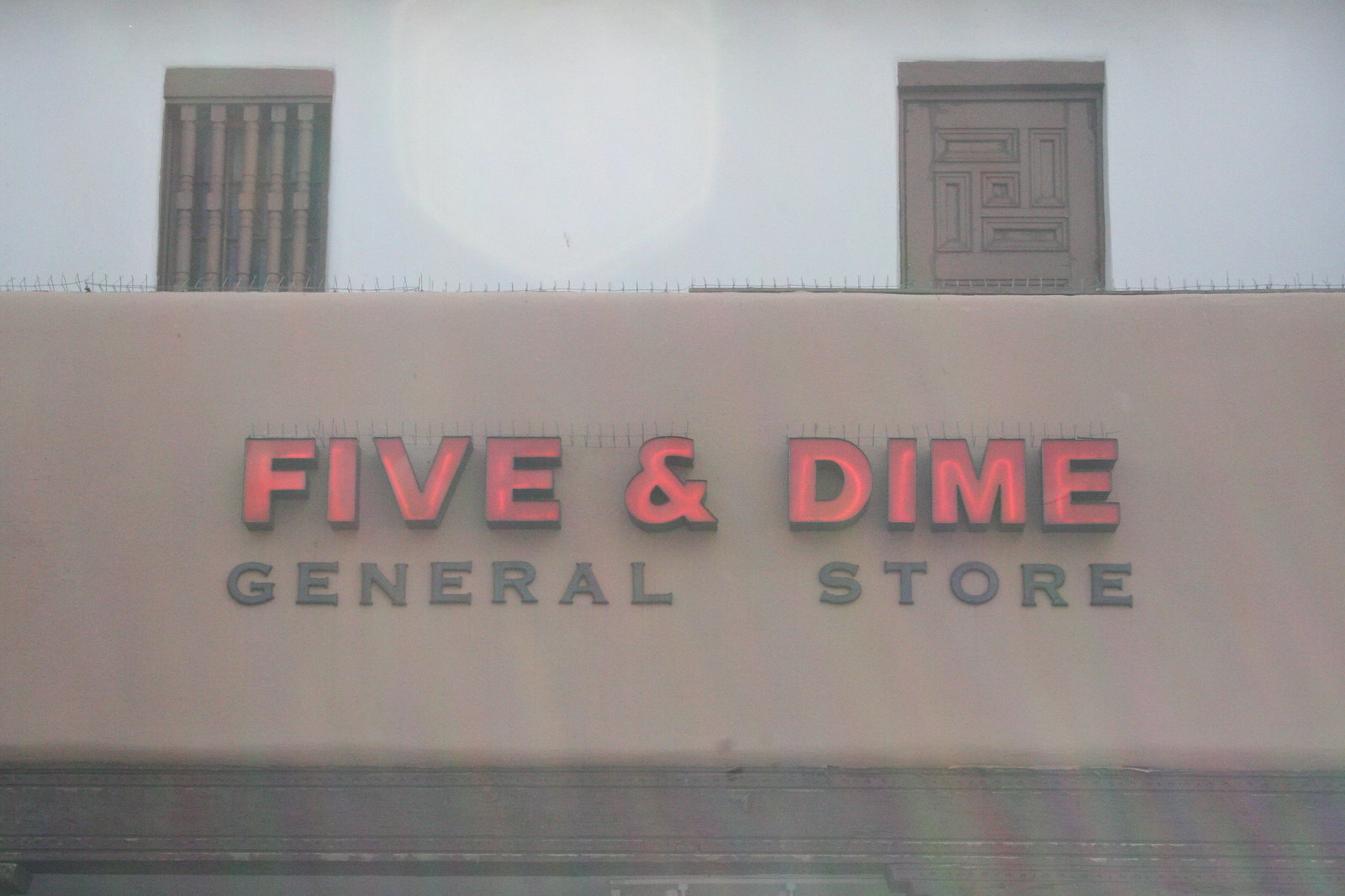This image captures the facade of a storefront featuring a rustic, vintage aesthetic. The building is primarily beige and beige-brown, with the store's name, "Five & Dime," prominently displayed in glowing red letters. The ampersand symbol is distinctly used in the signage. Just below this illuminating sign, the words "General Store" are written in a solid brown font. Above the signage, two intricate brown designs frame the top corners of the storefront, adding a decorative touch. Although their exact purpose is unclear, they resemble ornate windows or decorative grills. The image appears to be closely cropped, making it difficult to discern if the background above the sign is the sky or the top of the building. Below the signage, there is an additional brown strip, contributing to the overall earthy color scheme of the storefront.